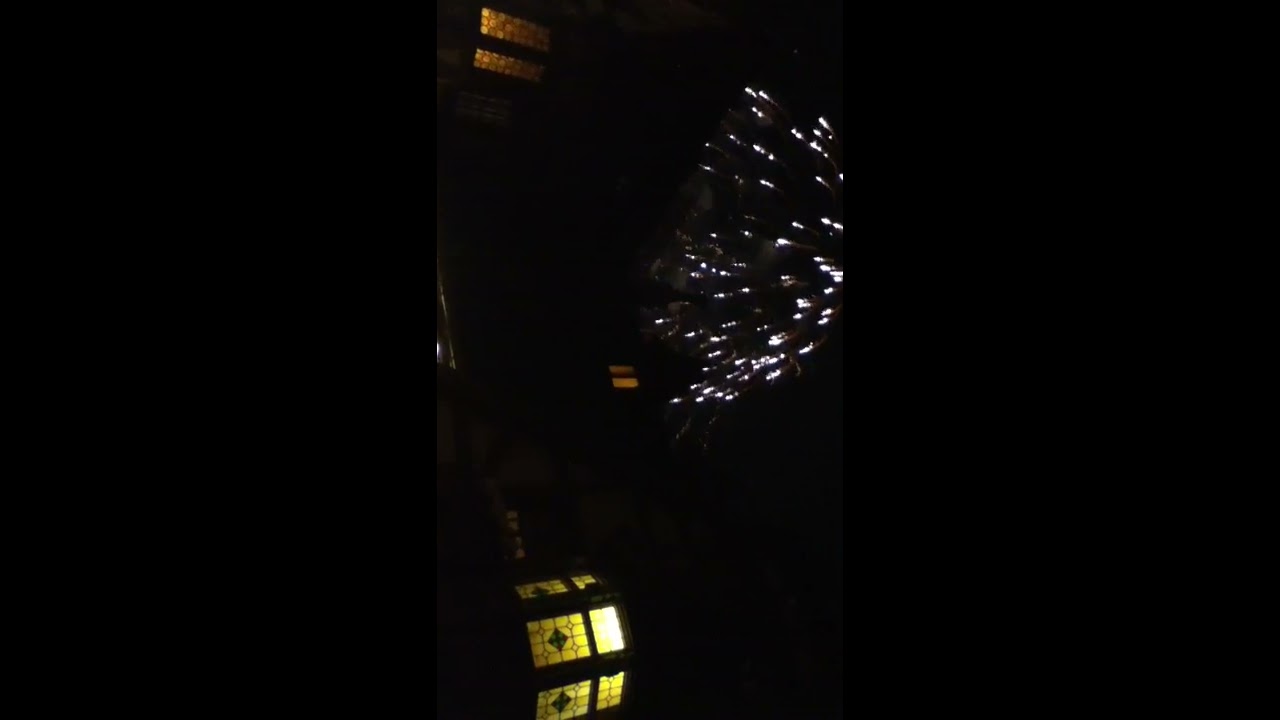This captivating color photograph, taken at night, is centered in a landscape-oriented frame with wide black borders. The central image, oriented sideways in a portrait layout, predominantly showcases a dramatic scene of phosphorescent white fireworks cascading downward, resembling a delicate mushroom shape. These bright, falling embers dominate the top left of the image. Below this spectacle, on the left side (which would be the bottom center if correctly oriented), faintly illuminated windows sit in an otherwise dark, empty neighborhood. These windows possess an ornate, stained-glass quality with intricate designs and hues of yellow, orange, and green, reminiscent of church windows. The light filtering through these opaque panes adds a touch of warmth to the scene's otherwise dark ambiance, providing a subtle but complementary background to the fireworks' brilliance.